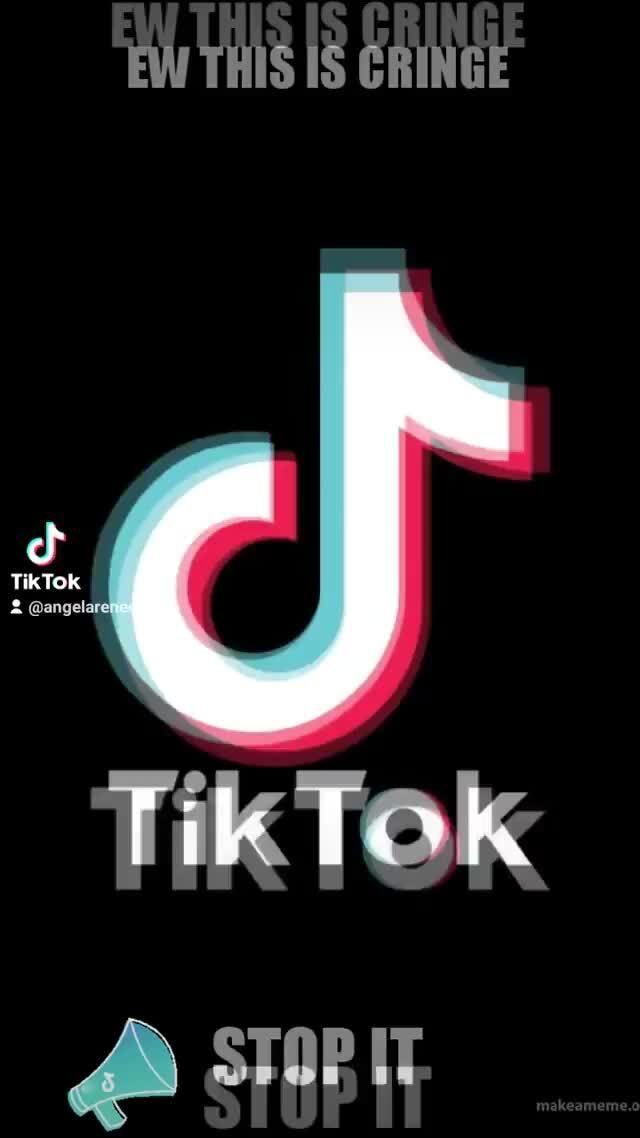The image is a vertically-oriented rectangle with a predominantly black background. At the top, in prominent white text, the phrase "ew, this is cringe" is repeated twice, creating an emphatic statement. Directly below this text sits the TikTok emblem, a well-recognized icon, with the word "TikTok" printed beneath it. Further down, in the bottom left corner of the image, there is a striking green megaphone graphic accompanied by the exhortation "Stop it." 

The bottom right corner subtly displays the mark of origin, "makeameem.com," barely perceptible against the dark backdrop. Each element in the image, whether it be text or graphic, casts a noticeable shadow, giving a layered and slightly three-dimensional effect. The duplication of the "ew, this is cringe" text, the TikTok emblem, and the "Stop it" phrase are all shadowed in this manner, enhancing the visual depth.

On the left-hand side, centrally positioned, there is another instance of the TikTok emblem with accompanying text, "at Angel Arena," repeated to reinforce the presence. This combination of elements provides a clear, detailed depiction of the meme, blending multiple text and graphic components with shadow effects for a visually engaging experience.